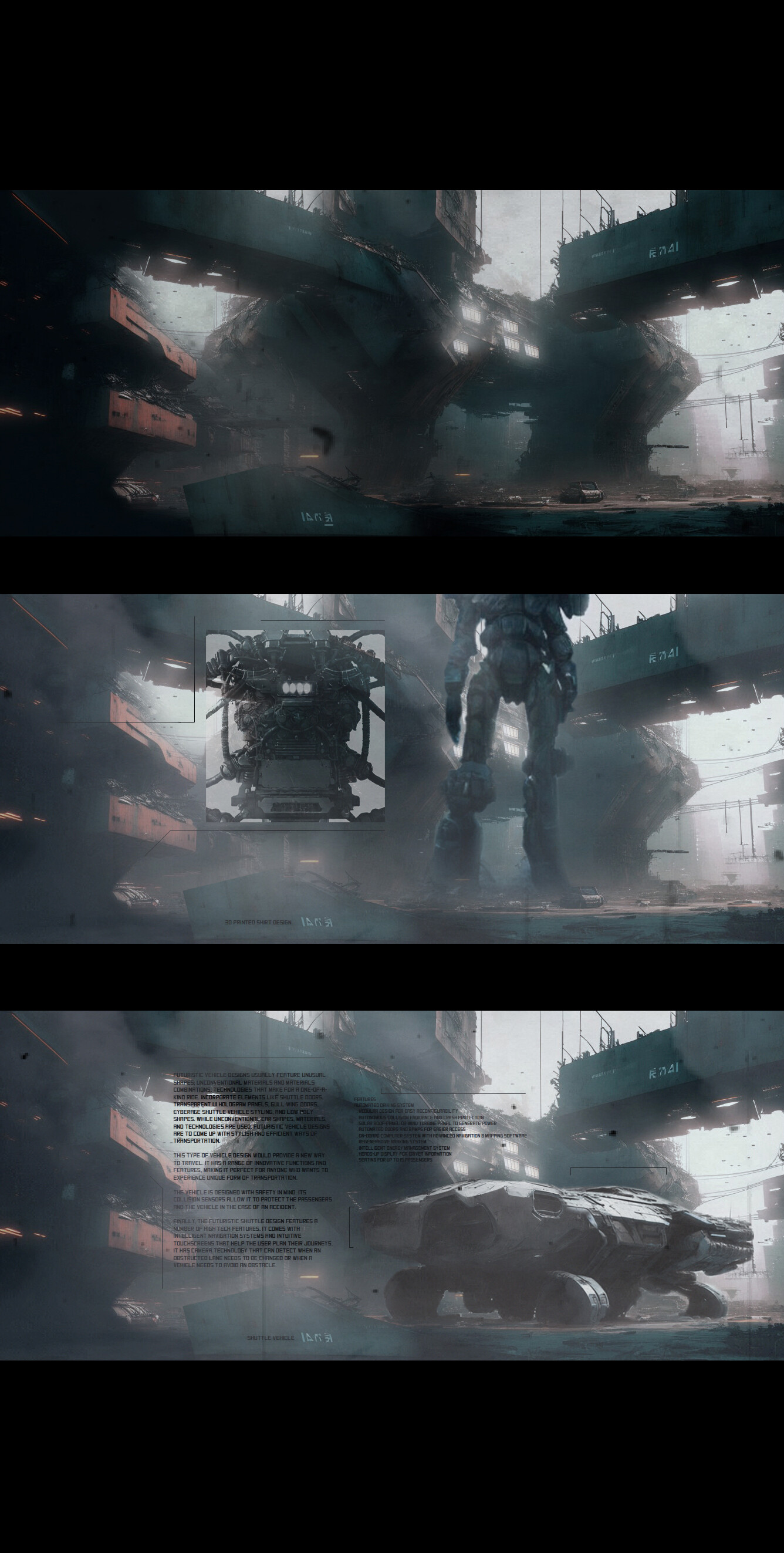This image features a vertically rectangular arrangement of three computer-generated scenes, with each frame divided by thin black horizontal borders and set against a black background, resembling a sequence of production stills from a futuristic video game or movie. The top image depicts a grainy and foggy industrial area, possibly a damaged bridge or construction yard, where indistinct structures and machinery loom amidst swirling dust. An open toolbox with two visible drawers sits to the left, hinting at ongoing, albeit unclear, activity. The middle frame shows a clearer view of the same industrial setting, with a large robot or humanoid figure in robotic armor standing on the right and a suspended motor on the left. The mechanical landscape is filled with metallic debris and gives off a sense of an abandoned or repurposed junkyard. The bottom image features a futuristic crawler robot with an insect-like appearance, positioned on the right. This frame also includes black text, difficult to decipher, superimposed over the chaotic industrial background, suggesting a narrative or technical details. The recurring elements and overall metallic, dystopian aesthetic of these frames evoke a vision of a bleak, mechanized future.